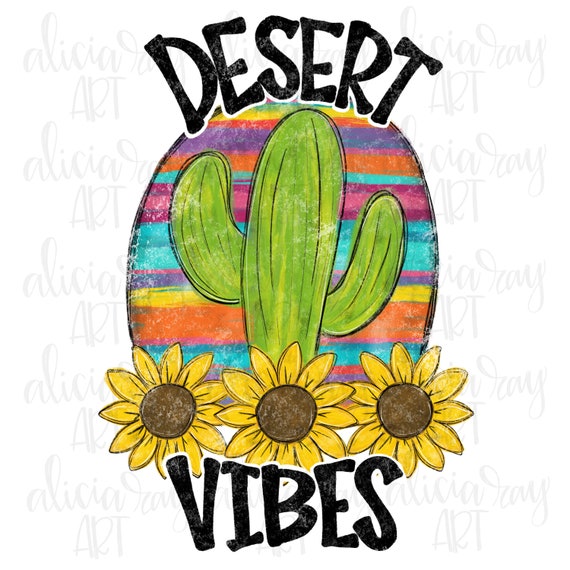This detailed description combines and emphasizes the shared and repeated elements from the three captions:

This image features a hand-drawn graphic design centered on a white background, which is subtly patterned with the watermark "Alicia Day Art" (or similar variations such as "Alice Alessia Ray Art") in a very pale blue, cursive, calligraphy-style font. Dominating the center of the frame is a rainbow-colored, horizontally-striated oval in vibrant hues of purple, orange, pink, and teal. Over the colorful oval, there is a prominent green saguaro cactus with a central column and two arm-like extensions. At the base of the cactus, three yellow daisies with brown centers are neatly lined up. At the top of the oval in a handwritten black font, the word "desert" is inscribed, while below the oval, the word "vibes" appears in the same handwritten style. The overall design, reminiscent of a vintage piece or a logo that might be found on a t-shirt, has a unique, slightly worn aesthetic, conveying a sense of nostalgic charm.